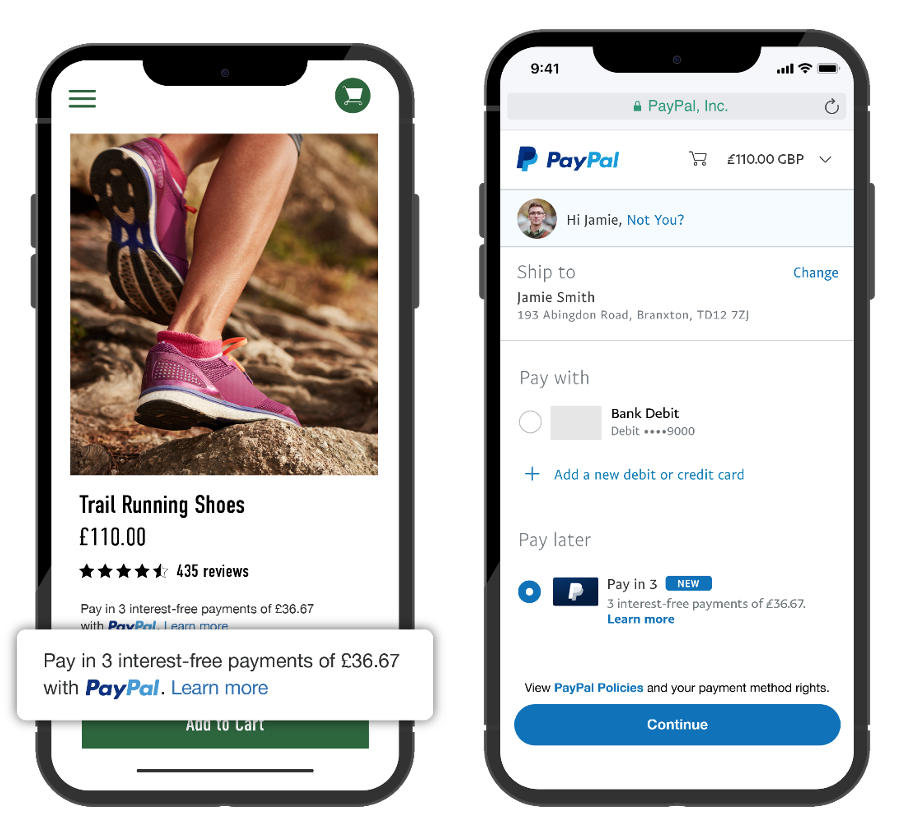Two cell phones are displayed side by side, both encased in sleek black covers, showcasing different screens. The phone on the left presents an online shopping app. In the upper right-hand corner, there is a shopping cart icon, while the upper left corner features three horizontal bars against a white background. The main image on this screen depicts a close-up view of a person’s toned calves, clad in vibrant purple running shoes, jogging over rocky terrain. Below this picture, bold black text reads "Trail Running Shoes" priced at £110. The item boasts a rating of four and a half stars from 435 reviews. Below the price, light gray text details a payment option: "Pay in three interest-free payments of £36.67 with PayPal. Learn more."

The second phone on the right has the PayPal app open. At the top is a search bar with “PayPal Incorporated” displayed inside it. Next to a shopping cart icon, the price of the selected shoes is visible. The screen greets the user with a profile picture of a young man and the text: "Hi, Jamie, not you?" Under this greeting, it states "Ship to Jamie Smith" followed by his address in light gray text. The screen offers two payment options: to pay with a debit card or through PayPal.